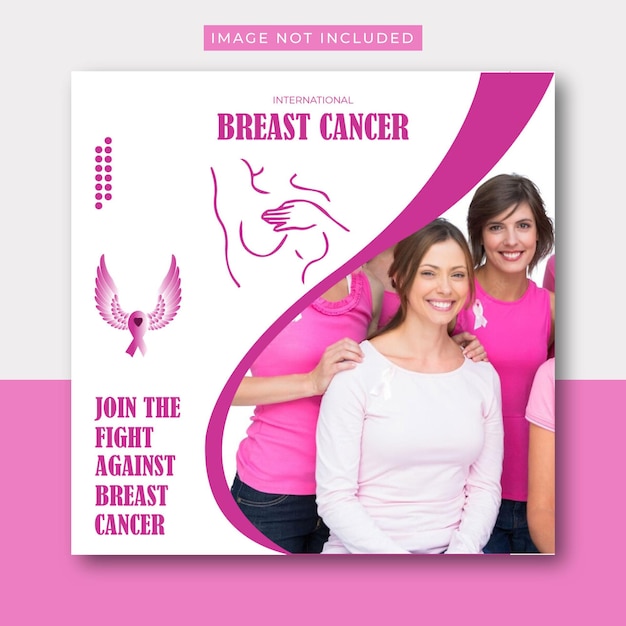The image showcases a computer screen with a predominantly square shape, featuring a gray background at the top and a pink background at the bottom. Positioned at the top center is a pink rectangle labeled "Image Not Included." Below this is a white, square-shaped box with a pink upper portion that reads "International Breast Cancer."

In the middle of the image, there is an outline of a female's body demonstrating a self-breast exam. Adjacent to this, on the bottom left, is a pink ribbon adorned with two eagle wings extending from its top, also in pink. "Join the Fight Against Breast Cancer" is prominently written in pink in the bottom left corner.

To the right of the text and outline, a pink banner separates this portion from another section of the image featuring several females. Two women are clearly visible: one is wearing a light pink long-sleeve shirt and has dark brown hair, smiling while someone places their hands on her shoulders. Behind her, another woman is dressed in a hot pink shirt with a pink breast cancer ribbon on the left side and has short brown hair. The remaining females are partially visible.